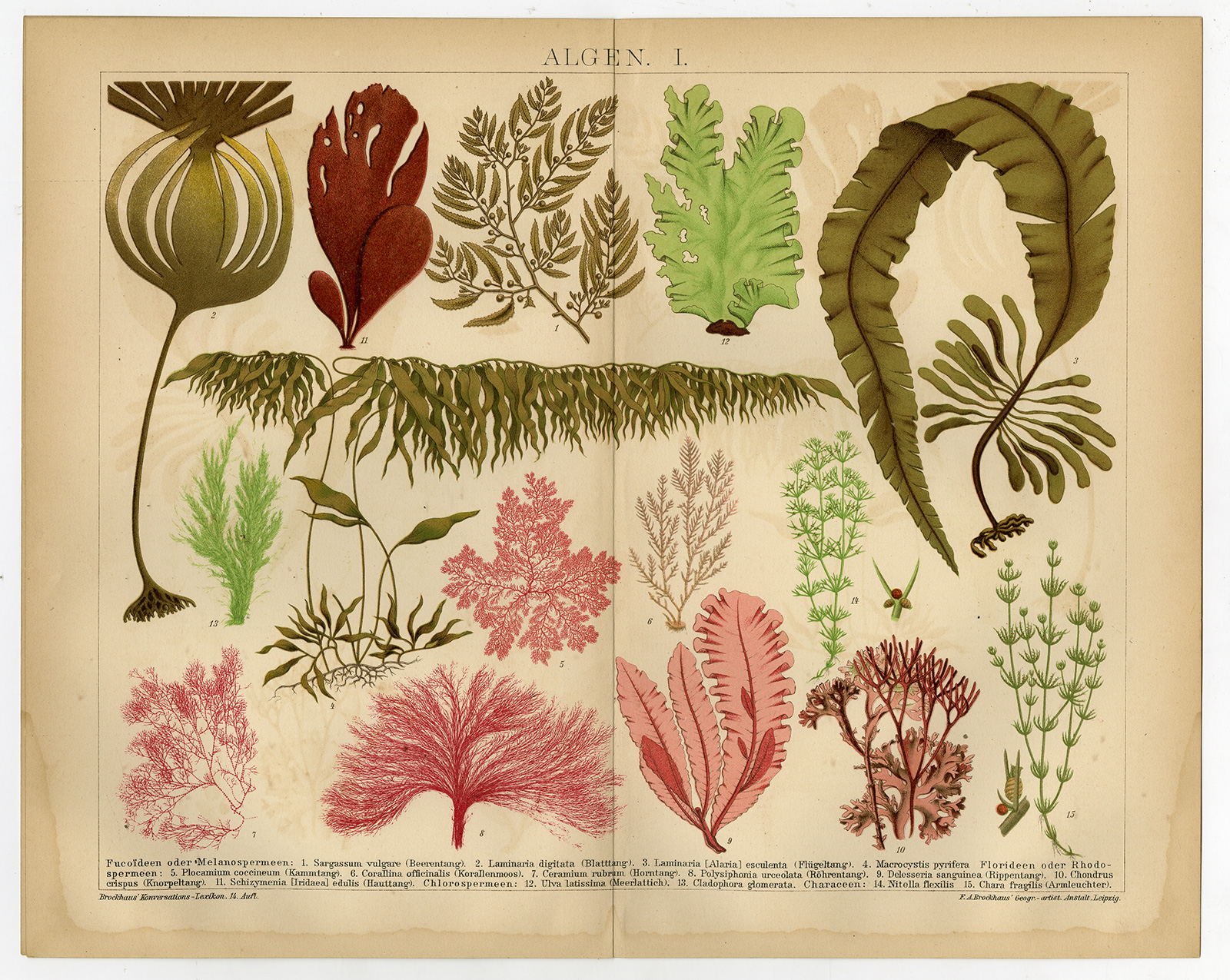The image depicts an open, older book illustrating various plant species. The top of the page prominently reads "ALGEN1" in dark letters. The open pages feature approximately 16 to 17 distinct plant designs, each meticulously detailed and numbered for identification. The illustrations showcase a range of plant parts, including fern-like leaves, small bushes, twigs, and larger sword ferns. The color palette is diverse, encompassing shades of green, pink, burgundy, maroon, yellow, red, gold, and brownish-gold. Notable among the plants is a large green leaf that curls at the top, a long green stem ending in a ball shape with numerous small offshoots, and several stems with thin, wavy leaves. Each drawing is carefully placed across the seam of the book, emphasizing the intricate details of each plant's structure.